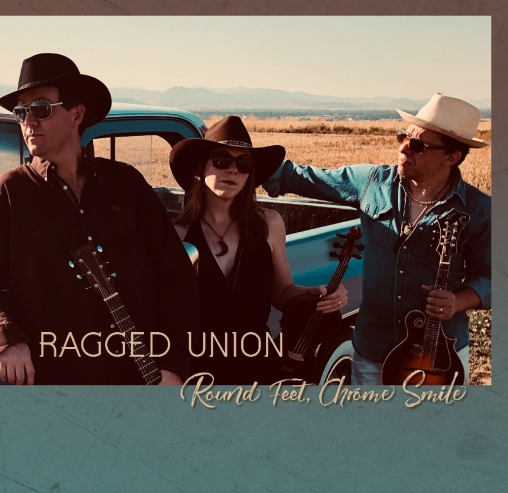This photographic image captures a trio of musicians posing against an old blue pickup truck in a picturesque desert or mountainous landscape. The setting is outdoors during the day, featuring a backdrop of brown bushes, distant buildings, and a mountain range under a light blue or gray sky. The three individuals, all wearing sunglasses and cowboy hats, exude a rustic charm, perhaps hinting at the cover of an album titled "Ragged Union, Round Feet, Chrome Smile," as indicated by the text on the image, highlighted by a blue border at the bottom.

On the left stands a tall white man in a black cowboy hat, navy sunglasses, and a long-sleeve brown button-up shirt, holding a full-sized guitar. The central figure, a woman, sports a brown cowboy hat and sunglasses, accessorized with a necklace featuring a distinct crescent moon pendant. She is clad in a v-neck vest and holds what appears to be a violin or small guitar. The man on the right, likely Hispanic, is seen in a white fedora, black sunglasses, a blue shirt, and light-colored pants, also cradling a small guitar or possibly a mandolin. The scene captures a harmonious blend of rugged individualism and musical unity, set against the tranquil yet rugged beauty of their natural surroundings.